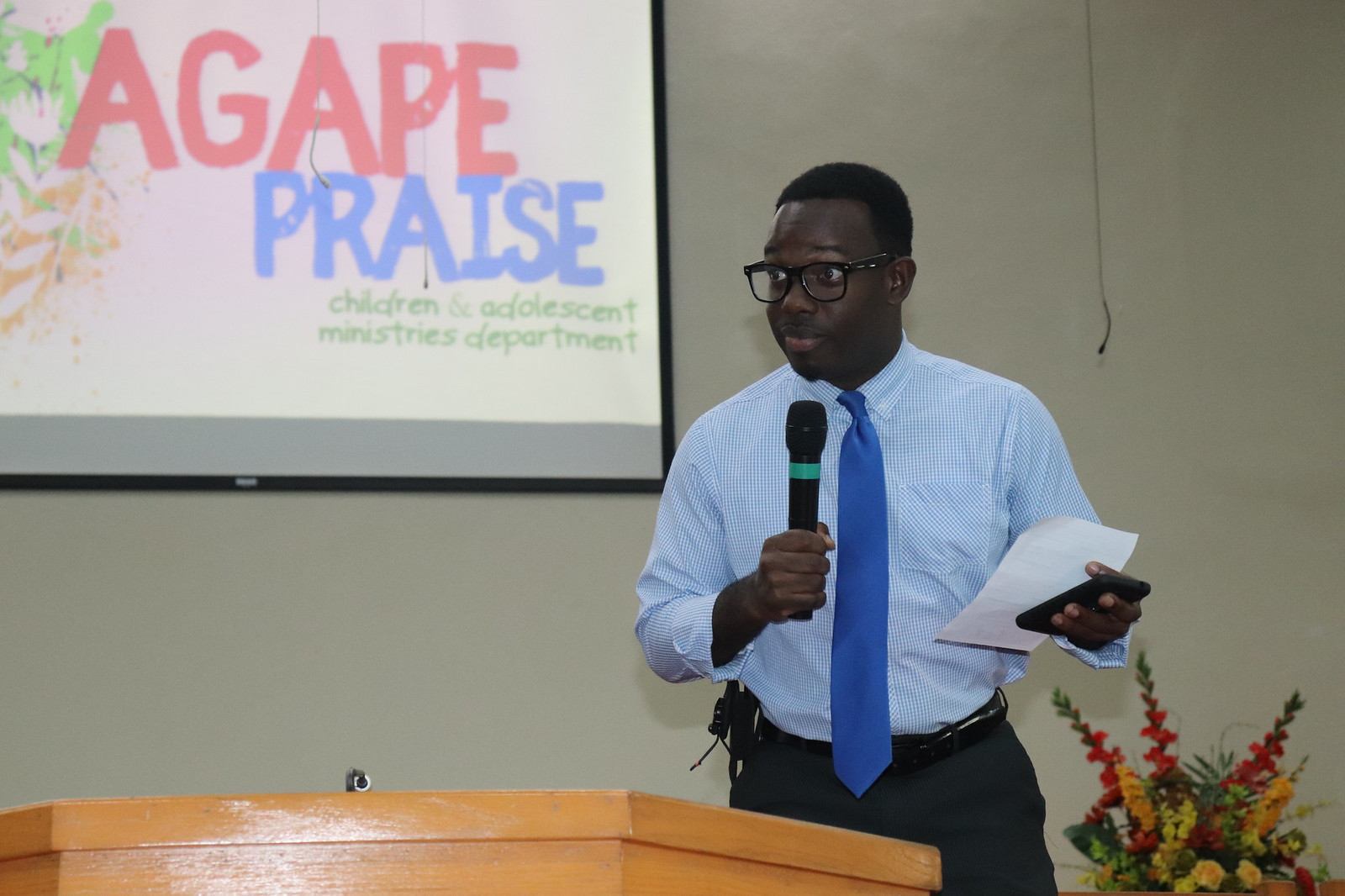This color photograph captures a well-dressed, dark-skinned African American man standing on a stage behind a wooden pulpit. The man, wearing black-framed glasses, presents a composed and professional appearance in a pale blue dress shirt with a medium blue tie, complemented by black slacks and a black belt. A battery pack or microphone is clipped to his belt on the right side. He holds a microphone in his right hand and a cell phone along with a piece of white paper in his left hand, suggesting he is in the middle of a presentation or speech. Behind him, a white wall hosts a projector screen displaying a colorful graphic that reads "Agape Praise, Children and Adolescent Ministries Department." To the man's right, at the bottom right of the photograph, a large and vibrant floral display adds to the setting's formality and warmth, indicating this might be taking place in a church, with the man possibly serving as a youth pastor.